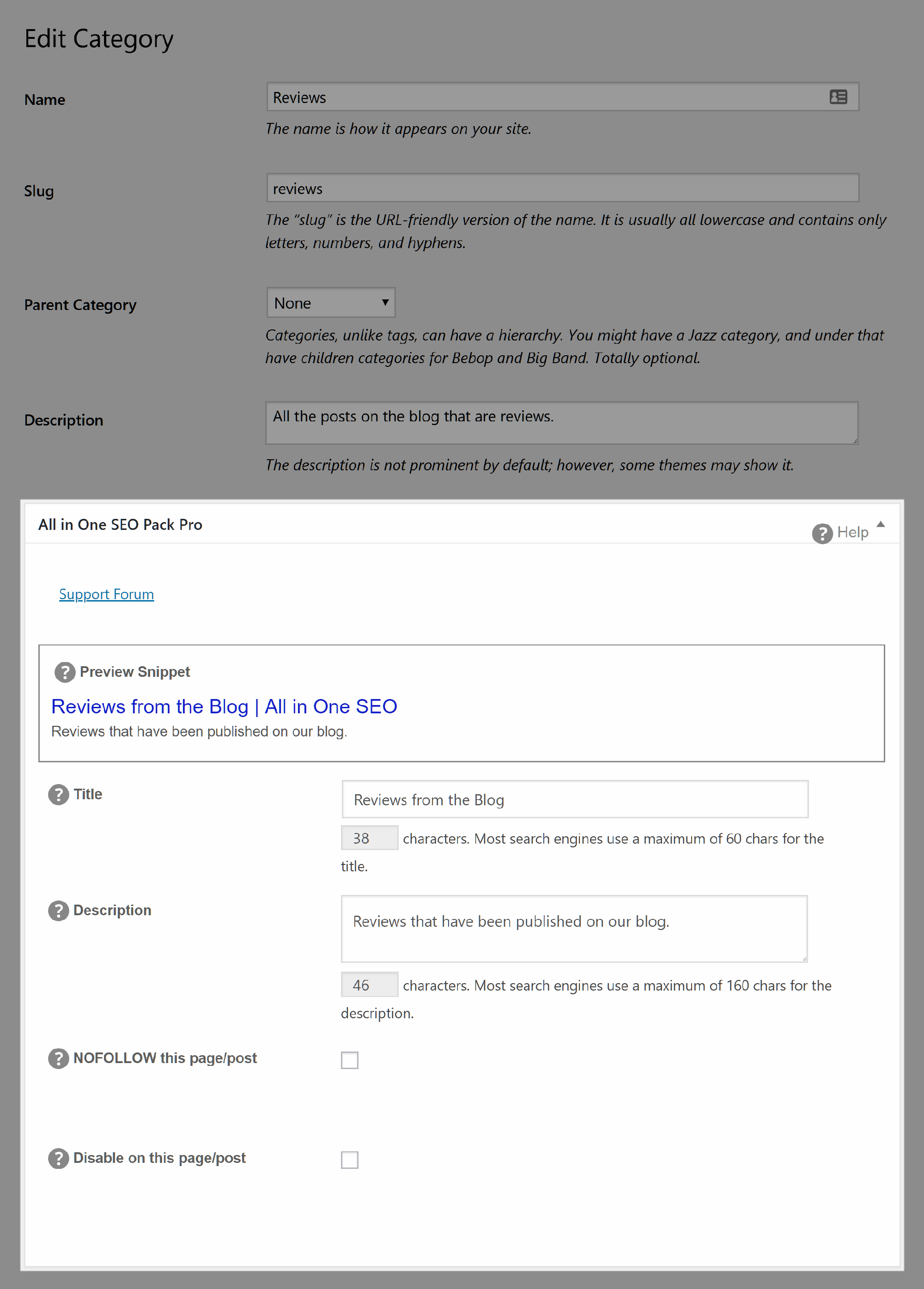An image showcasing a website interface featuring an open editor. The editor displays a preview of the "All-in-One SEO Pack Pro" tool with a darker background and a lighter foreground where editing is active. The editable sections include fields for the title, description, a checkbox to "No Follow this Page/Post," and a checkbox to "Disable this Page/Post." In the darker, non-selected background area, there are four labeled boxes for "Edit Category," "Name," "Slug," "Parent Category," and "Description." Specifically, the "Name" is set to "Reviews," the "Slug" is "reviews," the "Parent Category" is marked as "none," and the "Description" reads, "All the posts on the blog that are reviews."